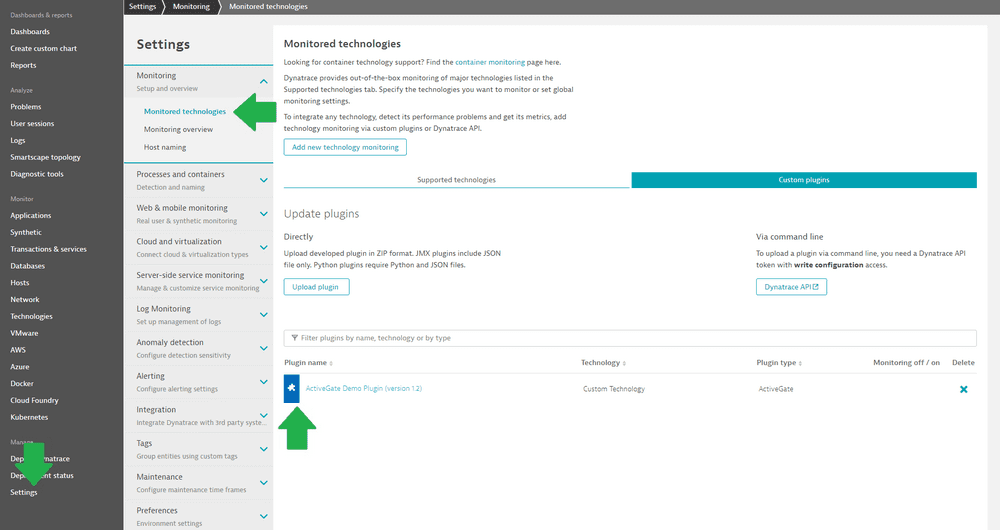The image captures a computer screen displaying a detailed dashboard interface for a monitoring application. 

In the top left corner, the section is labeled "Dashboard and Reports." Directly below this header, there is a vertical column listing various options: "Dashboards," "Create Custom Chart," "Reports," "Analyze," "Problems," "User Sessions," "Logs," "SmartScape Technology," and "Diagnostic Tools." 

Further down the interface, under a new section labeled "Monitor," additional text categories are displayed: "Applications," "Synthetic," "Transactions and Services," "Databases," and "Hosts," each followed by different sub-options.

The adjacent column on the right is titled "Settings" and includes subsections such as "Monitoring," "Settings," and "Setup and Overview." In this section, the text "Monitor Technologies" appears prominently in blue, accompanied by a large green arrow pointing towards it. The sub-options here include "Monitoring Overview," "Host Naming," "Processes and Containers," "Detection and Naming," "Web and Mobile Monitoring," and "Real User and Synthetic Monitoring". Additional text directs users seeking container technology support to find the "Container Monitoring" page.

Furthermore, the screen provides information that "Dynatrace offers out-of-the-box monitoring of major technologies listed under the Supported Technologies tab" and instructions to "Specify the technologies you want to monitor or set global monitoring settings." There is an option to "Add new technology monitoring."

Towards the bottom of the screen, it reads "Update Plugins directly," followed by an option to "Upload Plugin," accompanied by a corresponding button. Beneath this is a section titled "Plugin Name," where another large green arrow points upwards toward the text "ActiveGate Demo Plugin version 1.2."